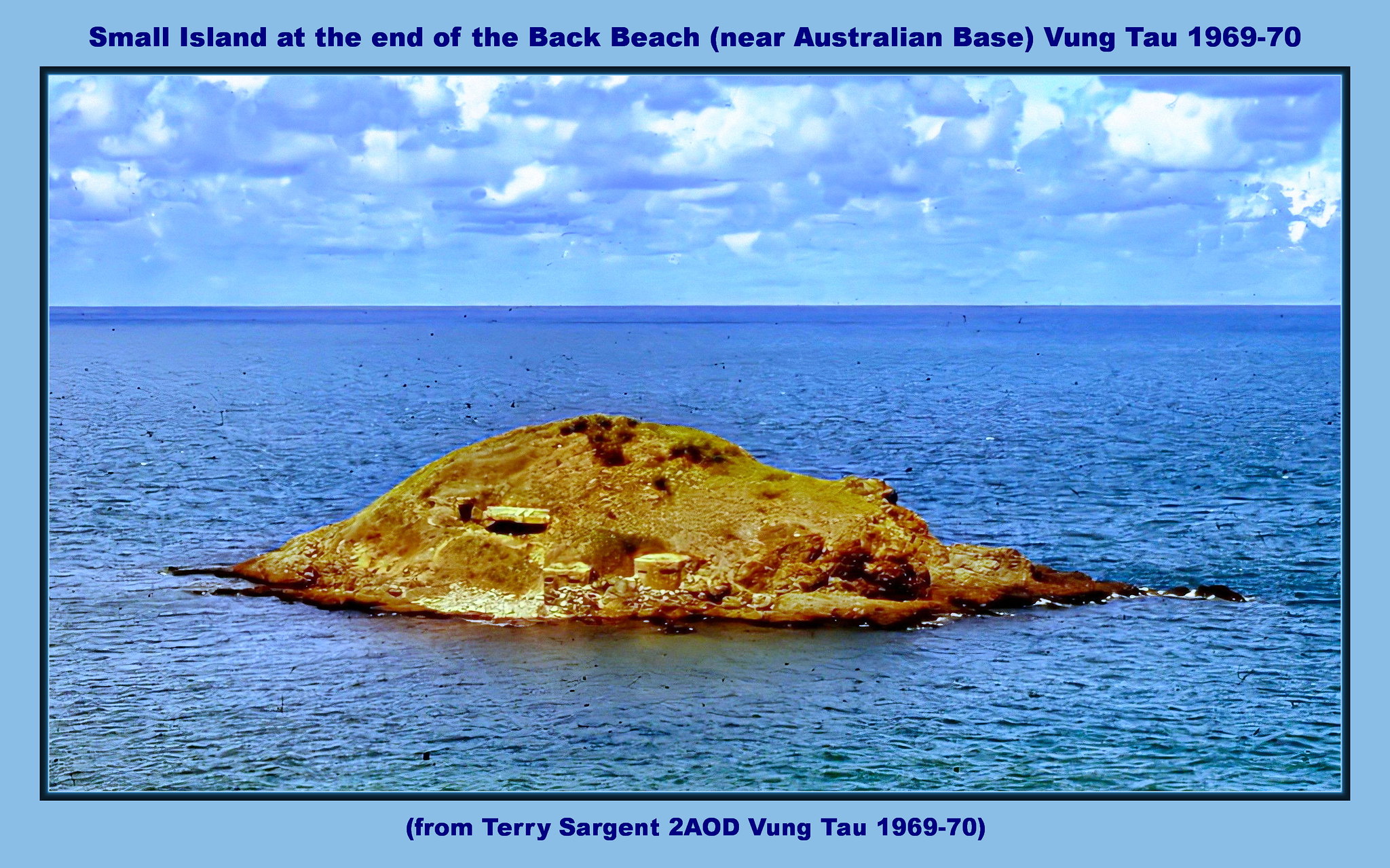The image is presented as a postcard with a horizontal rectangular photo set against a light sky blue background. The photograph within the postcard captures a serene sea landscape featuring a small island amidst calm, blue waters. The island is predominantly brownish-yellow, resembling a hill with patches of grass and rocks. There are what appear to be two cement structures or possibly old fortifications towards the center of the island. The sky above is mostly cloudy, interspersed with patches of blue and white, and a few birds can be seen hovering in the distance.

Above the photo, in dark blue text, it reads: "Small Island at the end of the Back Beach near Australian Base, Vung Tau, 1969-70." Below the photograph, it says: "From Terry Sergeant to AOD Vung Tau, 1969-70." The entire postcard maintains a blue theme with both the top and bottom captions in dark blue text, complemented by a light blue background and a smaller black border framing the image itself.